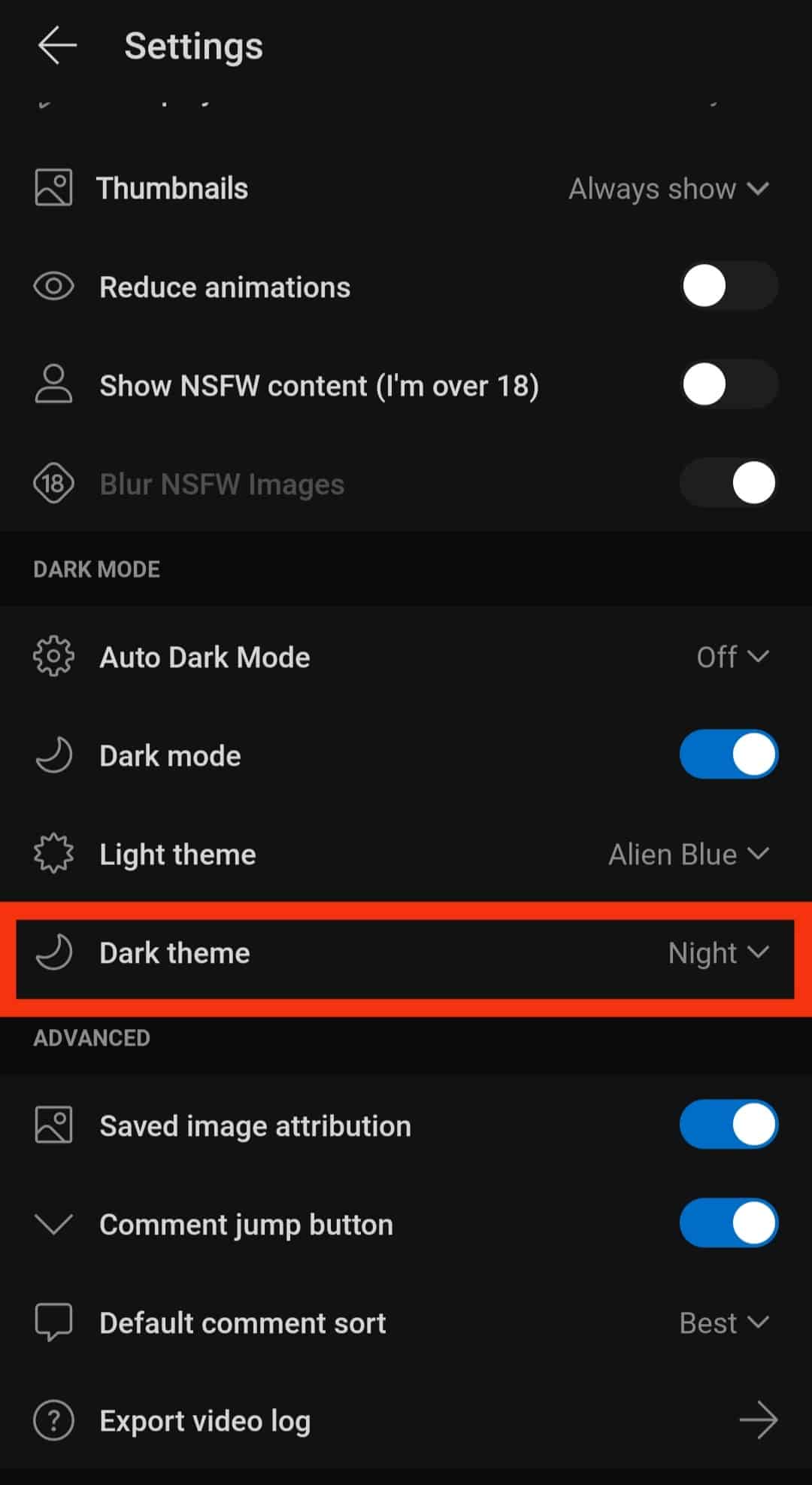A screenshot showcases a settings menu with a black background. At the top-left corner, there is a white arrow pointing left, labeled "Settings." The menu lists various options: "Thumbnails - Always Show," "Reduce Animations," "Show NSFW Content - I'm over 18," and "Blur NSFW Images - off." The theme settings are prominently featured: "Dark Mode - Auto Dark Mode - off, Dark Mode on, Light Theme - Alien Blue, Dark Theme - Night," with the "Dark Theme" section highlighted by a red rectangle. Additional advanced options are visible: "Saved Image Attribution - on," "Comment Jump Button - on," "Default Comment Sort - Best," and "Export Video Log," indicated by an arrow pointing right. The image is notably taller than wide, consisting entirely of text and interface elements, devoid of any photographic content, people, animals, or objects.